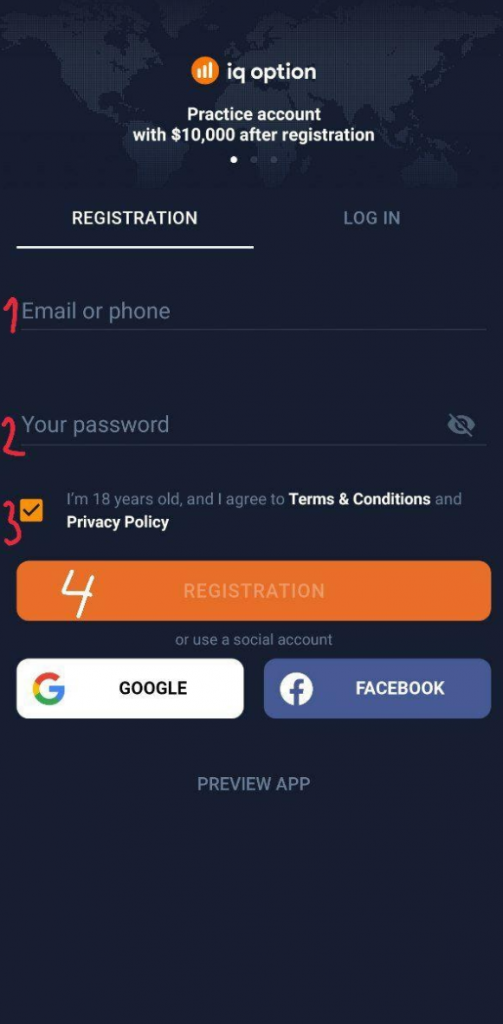A comprehensive description of the image would read: 

The image features a dark background providing a stark contrast to the other elements. At the top, 'IQ Option' is prominently displayed. Below this title, there is an orange solid circle containing a red saw and three bars, which symbolize the app's features. A significant portion of the image is occupied by a silhouette of the world map.

Directly below the map, there is a registration section beginning with the text "1. Registration". The steps are marked in a red font, making them stand out against the dark background. The registration process is divided into numbered steps with the first step labeled "1", followed by prompts for "Email or phone" and "Your password". 

Beneath these fields, there is a noticeable orange square featuring a black checkmark, with the accompanying text, "I'm 18 years old, and I agree to terms and conditions." Further instructions continue with the text "2. Registration" and the number "4". 

Additionally, the image highlights options to register via "Google" or "Facebook". At the bottom, there is a navigation element showing three dots, indicating that the screen can slide across three different pages. The final option on this registration interface allows users to "Preview the app."

The overall layout is designed to be user-friendly while emphasizing the registration steps and available login options, all set against a visually engaging and dark-themed background.